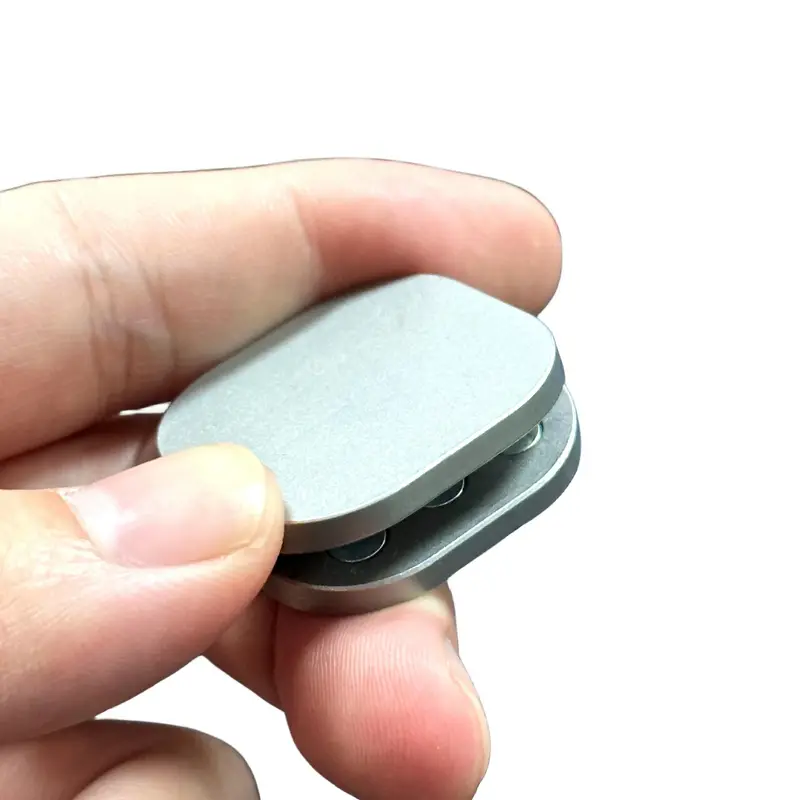The image features a close-up of a well-manicured hand delicately holding a small, silver metal device against a clean, white background. The hand appears to be from a white individual and is strategically positioned to highlight the product. The index finger is straight, gently resting on the top edge of the device, while the thumb secures the bottom right corner. The middle finger is curved beneath the device, providing additional support. The metal device itself has a dull, matte finish and is square-shaped with rounded corners. It is slightly open, revealing a dark gray interior with three partially visible circular shiny spots, which resemble screw heads. Embedded inside are magnets, ensuring that the two pieces of the device lay flush when closed. The simplistic white backdrop enhances the focus on the hand and the device, suggesting that the image is likely for promotional purposes to sell the product.